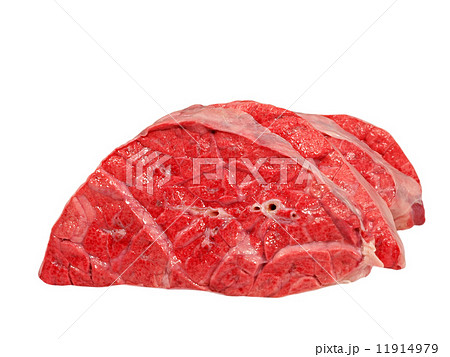The image depicts three slabs of very fresh-looking meat, each exhibiting a deep red color with varying shades of yellow, white, and gray fat marbled throughout. The meat's texture has prominent ridges and curvatures, suggesting it could be either ground beef or a cow's brain, adding to its intricate, organic appearance. Over the surface of the meat, a clear plastic-like film is visible with gray lines angling towards the center. Small black holes encircled in white add further detail to the central section. The image features a watermark, with the text "PIXTA" faintly seen on the left side amid three identical arrows pointing left, and repeated more prominently in white at the top center. In the bottom right corner, "PIXTA.jp-11914979" is printed in black or gray, identifying the source as a stock image. The white background further enhances its clinical, clipart-like presentation.